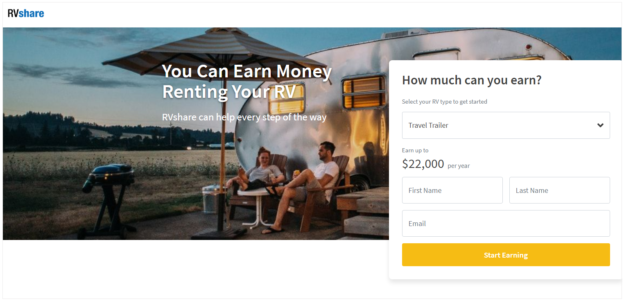The image captures a serene evening scene featuring a couple relaxing in rocking chairs under an umbrella, with their feet up. The backdrop showcases their RV, suggesting a peaceful, mobile lifestyle. To the left of the couple is a barbecue pit, adding a cozy, homely touch to the setting. The sky indicates it's dusk, adding a warm, tranquil ambiance to the scene.

A prominent header at the top reads "RVshare" with "RV" in bold black and "share" in blue lowercase, emphasizing the service. A text box explains that RVshare helps people earn money by renting out their RVs and provides assistance every step of the way. Another pop-up box prompts users with "How much can you earn?" and guides them to select their RV type, starting with a travel trailer. It specifies that a travel trailer can earn up to $22,000 a year, but requires first and last names along with an email address to get started. The call-to-action is highlighted with a white text on an orange button saying "Start Earning."

The overall design is clean and straightforward, making it easy to understand the service being offered. The highlighted image of the couple enjoying their time brings the concept of RVshare to life, emphasizing the joy and freedom it offers.